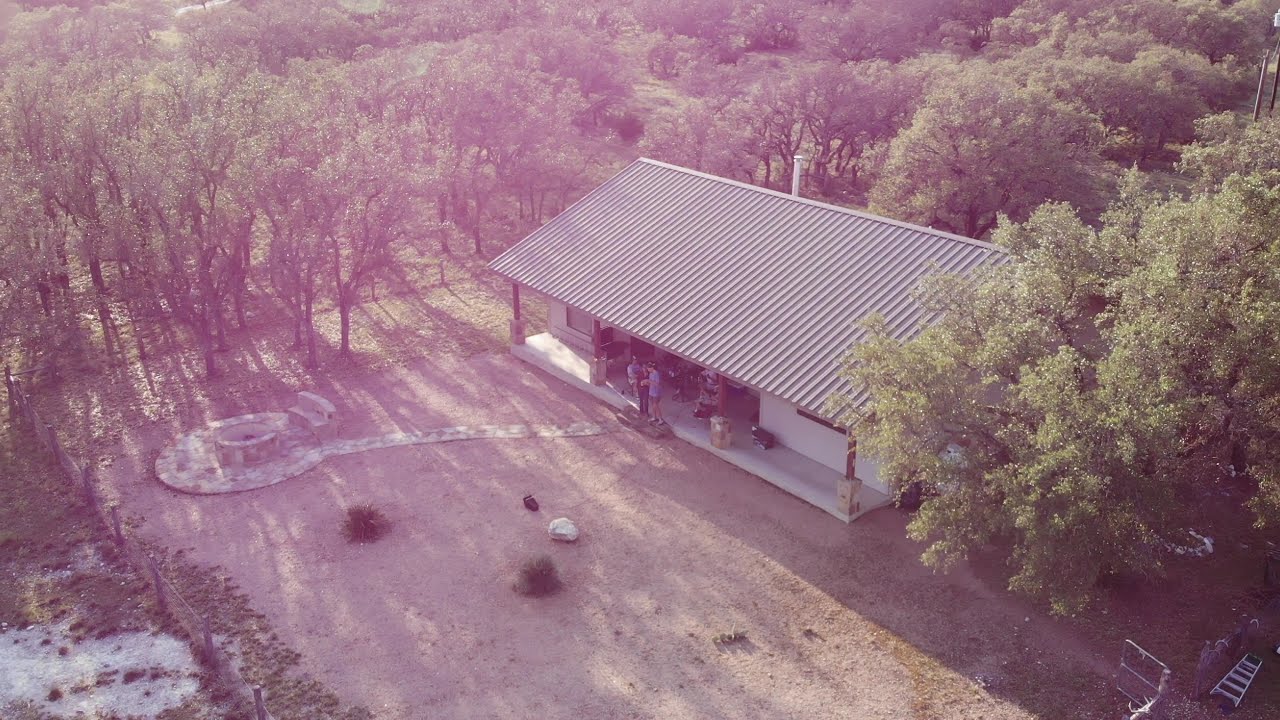This overhead image captures a one-story residence nestled in a wooded area. The property features a corrugated steel roof and white exterior walls, set upon a concrete slab. The roof slopes low with a prominent chimney stack in the center. A cement porch stretches along the front of the house, supported by pillars. In front of the house, a circular stone path leads to what appears to be a wishing well, surrounded by a gravel parking pad. Scattered around the property, the land is mostly dirt with some grassy patches and a white bench situated on the stone path. There are several people standing near the entrance—one dressed in a blue shirt and shorts, another in dark clothing, and one in a white shirt. The yard is enclosed by a silver fence, and a silver ladder lies on the ground at the bottom right corner of the image. Shadows indicate that the photograph was taken on a sunny day, although the overall scene is somewhat dark, casting some areas in deeper shadow. The surrounding trees, with brown trunks and green leaves, provide a dense and private setting for the home.